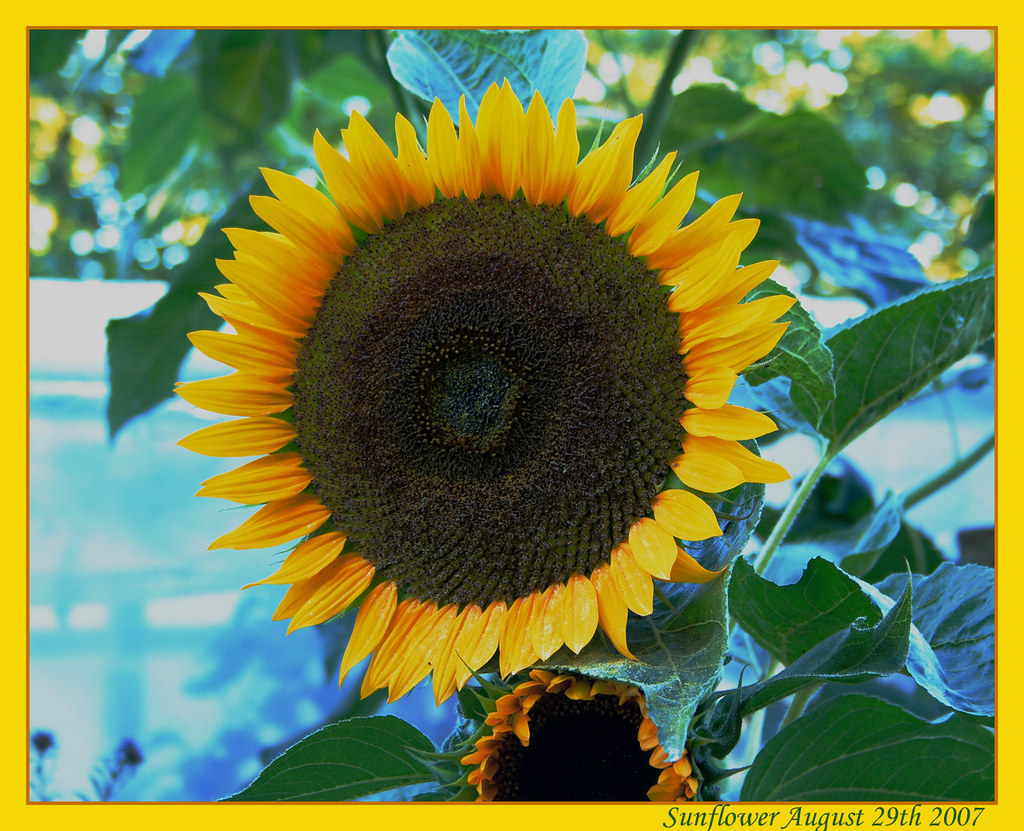The photograph taken outside on an overcast day showcases a vibrant sunflower in full bloom as the focal point. The sunflower, oriented slightly to the left, displays a captivating gradient of petals transitioning from dark orange near the center to bright yellow at the tips. The central disk of the flower features a mix of brown, green, and black hues. Surrounding the sunflower are lush green leaves, and beneath it, a smaller, not fully bloomed sunflower can be seen. The blurred background hints at indistinct trees and possibly a house, adding depth to the image without detracting from the sharp focus on the sunflower. Encasing the photo is a dual-colored border, consisting of a thin orange inner border and a broader bright yellow outer frame. At the bottom right, the caption in green font reads, "Sunflower, August 29, 2007."